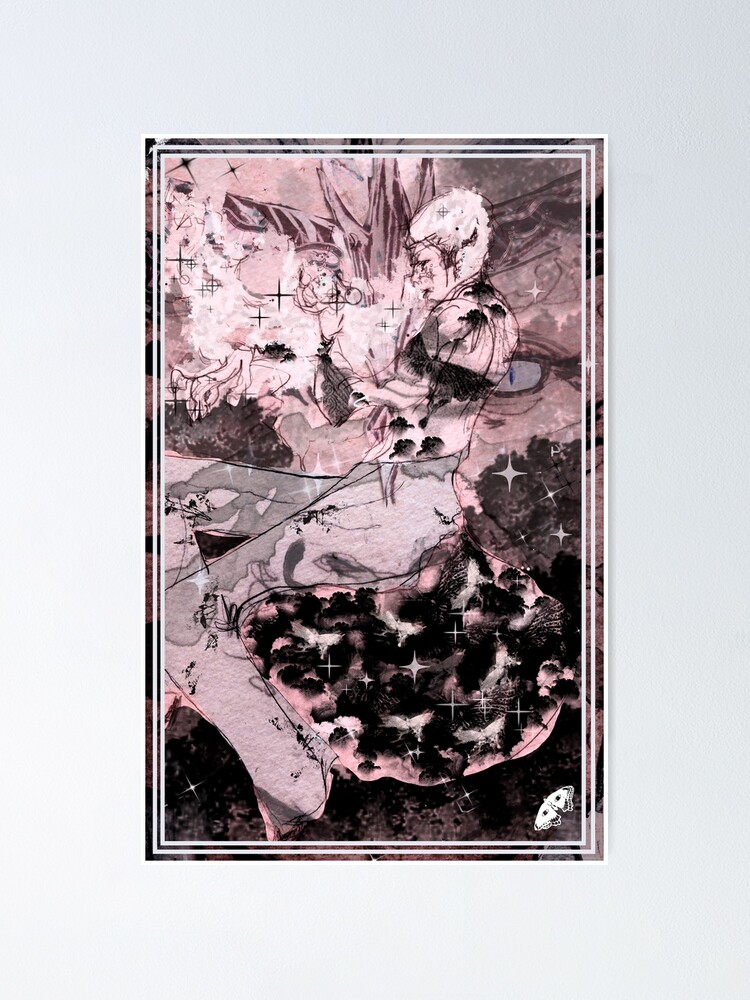The image depicts a vertically oriented, rectangular abstract illustration that features a double white inner border and a thin white outer border. The artwork is a chaotic blend of swirling lines and vibrant colors, predominantly black, pink, cream, and light purple. Within this colorful maelstrom, in the top right corner, one can just discern the left side of a woman’s face, which is turned towards the lower left hand corner. She has short or pulled-back blondish hair and is wearing a short-sleeved shirt featuring a swirling pattern of black and grayish cream hues. The abstract nature of the drawing obscures further details. 

In the lower right corner, there's an ambiguous object resembling a space vehicle with wings against a dark background, while a star is visible in the lower left corner. The central portion of the illustration suggests a figure, possibly sitting on a rounded rock-like object, with white hair and a shirt adorned in white, black, and purple hues. Above the figure's head, spiked purple lines extend towards the top of the image, and scattered black crosses appear in the upper left corner. The overall chaotic composition and brush strokes create a busy and intriguing visual. The image rests against a solid light gray background, making the eclectic colors and forms within the artwork stand out vividly.